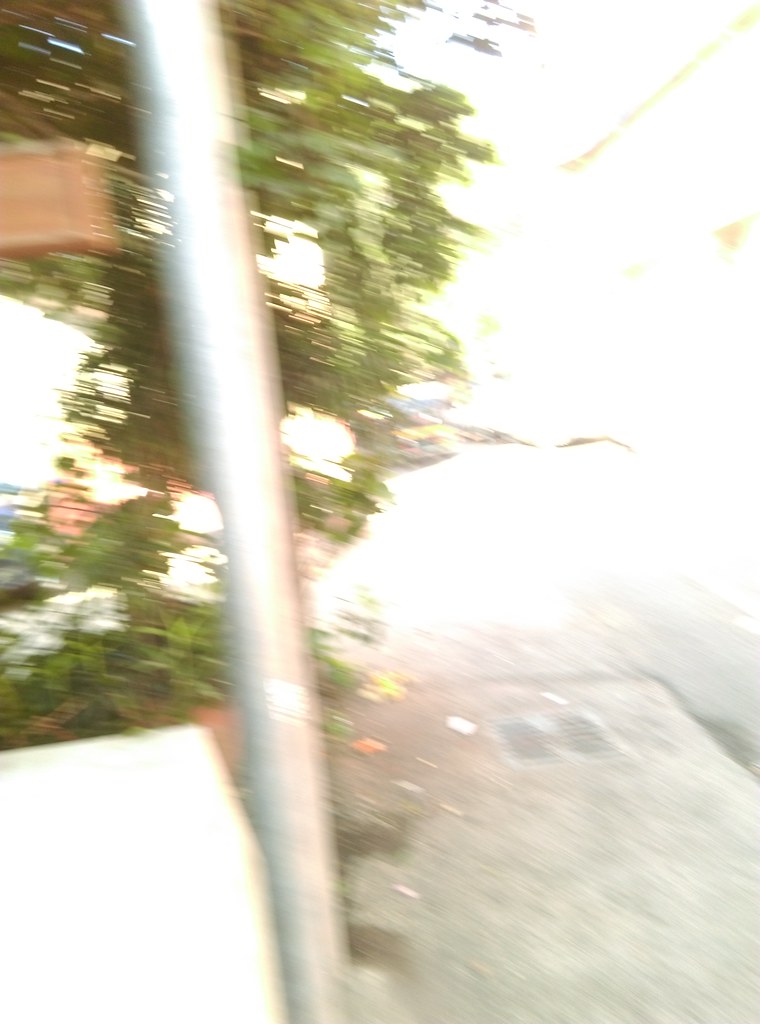This photograph features an extremely blurry scene, most likely captured while the camera was in motion, creating horizontal streaks across the image. In the foreground, a slender aluminum metal pole angles from the top left corner to the left middle of the image bottom. The pole is set against a backdrop of indistinct green streaks, suggesting foliage from a tree or shrub. To the left of this pole are some blocky shapes in brown and white hues, while to the right, the backdrop is stark white, indicating a strong glare from bright natural light on a sunny day. Below this, the concrete surface of the sidewalk is visible, with a drainage grate located towards the bottom two-thirds of the image. The image gives off a sense of a bus stop or similar urban setting, with occasional hints of yellow lines and potential asphalt adjacent to the sidewalk.